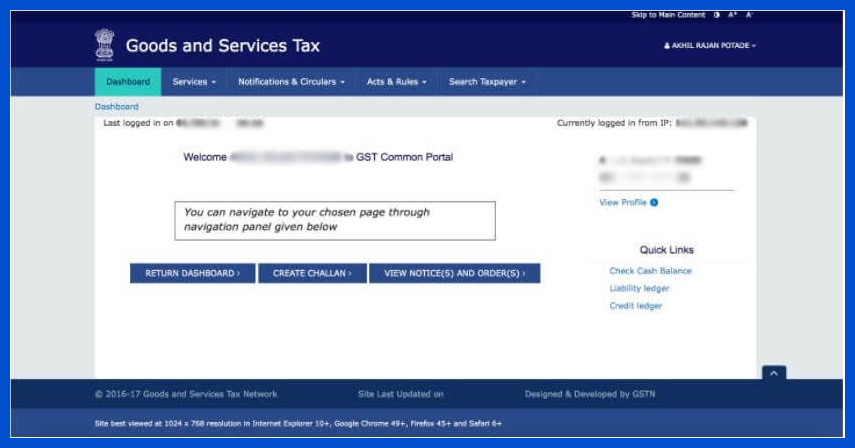A detailed screenshot of a window with a prominent blue outline features an engaging user interface for a "Goods and Services" page. The window itself is accented by a blue header, which prominently displays the title "Goods and Services" next to a logo on the left. To the right of the header, the profile name "Akhil Elajian Potade" is shown. 

Directly beneath the title is a well-organized menu bar with tabs labeled "Dashboard," "Services," "Notifications and Circulars," "Acts and Rules," and "Smart Taxpayer." The user interface also includes a breadcrumb trail starting with "Dashboard," and located below this is a large white information box. The white box contains a welcome message (with some content redacted) and is titled "GST Common Portal."

An italicized, boxed section within this white box provides navigation instructions: "You can navigate your chosen page through the navigation panel given below." Below this instruction are three blue buttons aligned in a row: "Return to Dashboard," "Create Chalan," and "View Notices and Orders."

On the right side of the interface is another section labeled "Quick Links," which lists three links: "Check Cash Balance," "Liability Ledger," and "Credit Ledger." A note about the current login IP, partially redacted, is displayed in the top right corner.

The overall layout and design elements of this page aim to facilitate ease of navigation and user engagement in managing goods and services transactions.